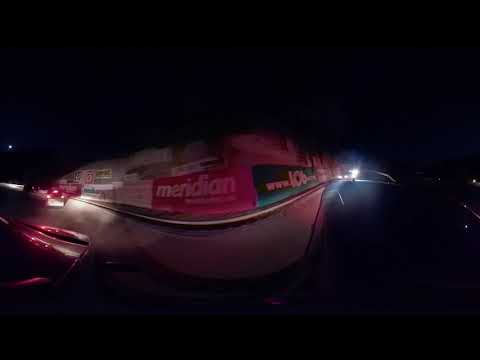The image captures a dark, nighttime street scene with a curved road section. The majority of the view is enveloped in deep shadows, both in the upper and lower halves. In the center, there's a brightly lit curved wall adorned with various signs and banners, creating a striking contrast against the darkness. The most prominent sign reads "meridian" in all lowercase, displayed in bold white text against a red background. To its right, another sign features the URL "www.i06.com" in white text on a green background. Two additional signs are to the left of "meridian", but they are too blurry to decipher, and there appear to be two or three more signs above it, though these too are small and unclear.

On the left side of the image, a car is driving away, distinguished by its visible brake lights. Directly above it is another car. Nearby, a white car is discernible by its three lights: one on each end and one on top. Behind this white car, there appears to be a black truck. On the right side, a car approaches, characterized by its white headlights shrouded in the overall dark ambiance. The entire scene seems to be viewed from a car or a building, adding a sense of perspective to the mysterious and dimly lit street. The curved layout of the image suggests it may be a result of panoramic photography, emphasizing the elongated and somewhat distorted view of the street and signs.